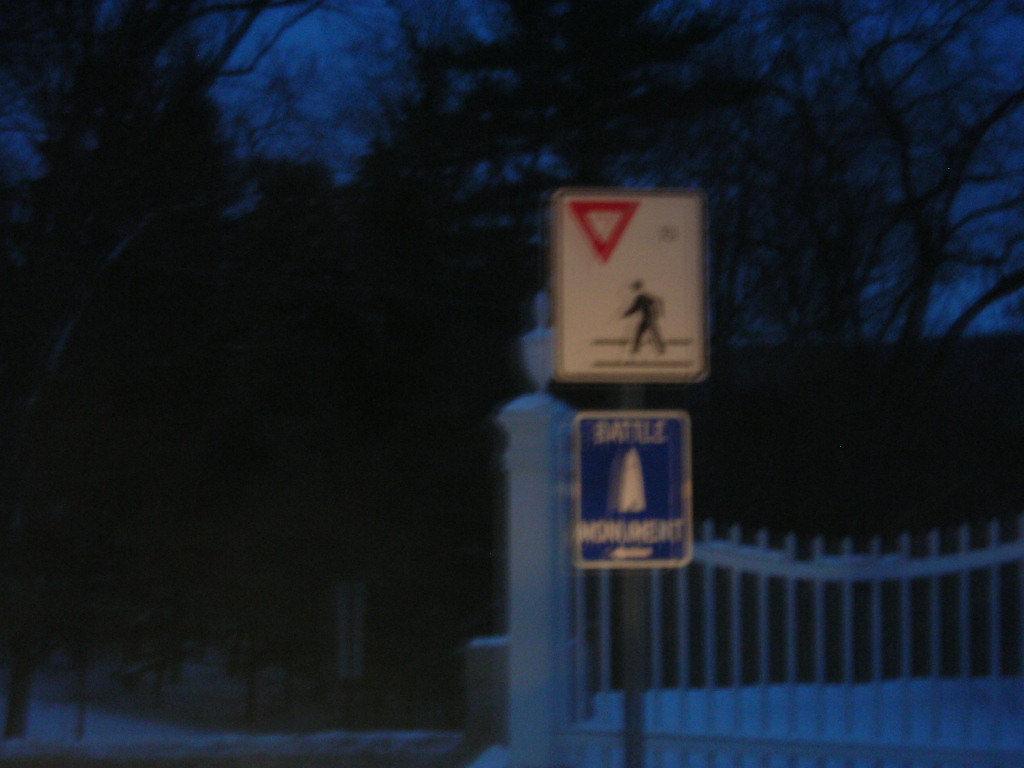In this atmospheric and slightly blurry photo taken outdoors at either dawn or dusk, the sky exhibits a dark bluish-black hue. Surrounding the sky are the silhouettes of barren, skinny trees without leaves, partially obscuring the view and adding to the scene's eerie tranquility. The foreground features an elegant wrought iron fence painted in white. This fence subtly curves, with a decorative fixture or shield design adorning the top of its large left post. Mid-ground is a dual-sign post: the top sign, primarily silver, displays a red downward-pointing triangle indicating "Yield," along with a pictogram of a stick figure walking in a crosswalk, directing drivers to yield to pedestrians. Below it, a blue sign with a white border and illegible white text, potentially reading "battle monument" with a leftward pointing arrow, stands prominently. The faint glimmer of snow at the bottom of the image hints at a cold, wintry setting, encapsulating the serene, softly lit scene.